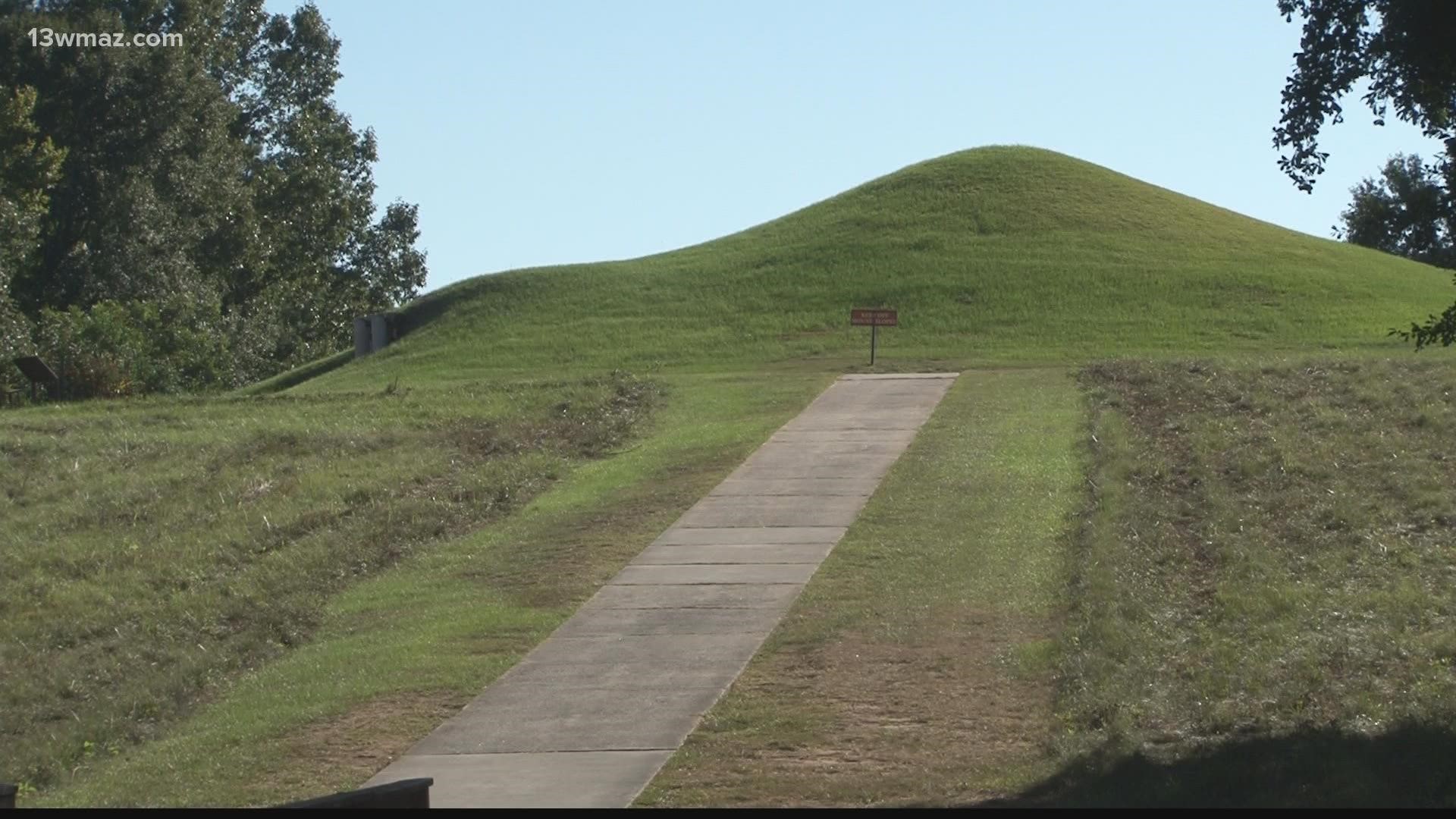The photograph captures an outdoor scene in the daytime, likely a section of a park or a historical site. Central to the image is a gray concrete walkway that extends from the bottom center straight up towards the background, leading to a neatly manicured green hill devoid of trees. Along both sides of the pathway, the grass varies in appearance, with some patches adjacent to the path turning brown, while the further outer sections appear more untamed. At the end of the walkway, right before the hill starts, there is a small brown sign on a pole that features white text that is too distant to decipher. The left upper quadrant of the image features a large, dark green tree, while the upper right quadrant reveals parts of another tree. The sky above is clear and light blue, providing a serene backdrop. Additionally, there is a line of text at the upper left of the image reading "13wmaz.com," hinting at a possible source or related site.